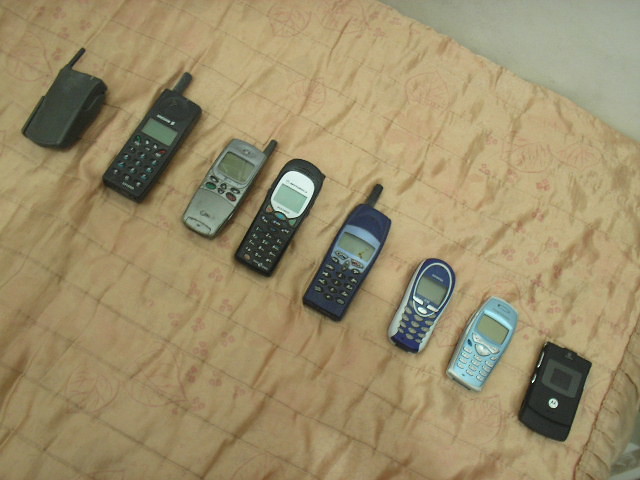The image displays a collection of eight old-fashioned cell phones from the early 2000s, arranged on what appears to be a tan, cloth-like bedspread. Notably, these phones vary in design and functionality, representing a nostalgic array of mobile technology from that era. 

On the far right, a black Motorola Razr flip phone stands out, reminiscent of the popular silver model from that time. Moving left, two candy bar-style Nokia phones are included, renowned for their indestructibility. Central to the arrangement are two Motorola phones; one is a black candy bar phone with exposed keys, and the other is a gray/silver phone featuring a fold-out flap concealing its buttons. 

The leftmost section includes a mix of less identifiable, potentially unbranded phones, further emphasizing the diversity in design. Among these, there's a black flip phone with a stubby antenna, a black slab phone, and a light blue candy bar phone with silver sides and buttons. Additionally, a dark blue candy bar phone with a stub antenna is present.

The majority of these devices are standard cell phones with a numeric keypad and call buttons, with approximately half featuring a stubby antenna while the others have an integrated antenna. This diverse collection epitomizes the mobile phone technology prevalent in the early 2000s.